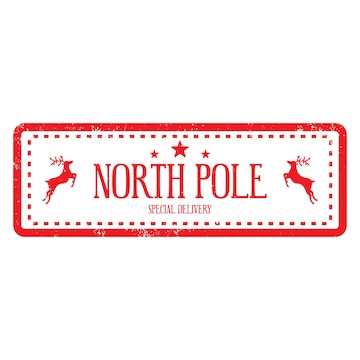The image depicts a rectangular sign with a distinct red and white color scheme. The background of the sign is white, while a solid red border encompasses the entire image. Inside this border, there is a second, inner frame made up of dotted red lines, encasing the central design elements. At the top center of the sign, there is a large red star flanked by two smaller red stars, creating a symmetrical arrangement. Prominently displayed in the middle of the sign is the text "North Pole" in bold red letters, and just below it, in smaller red text, are the words "Special Delivery." On either side of this text, there are reindeer figures, both in red, depicted with their front legs raised as if prancing. The overall design is simple yet striking, evoking a festive, holiday-themed logo or stamp with a clean, uncluttered white background.